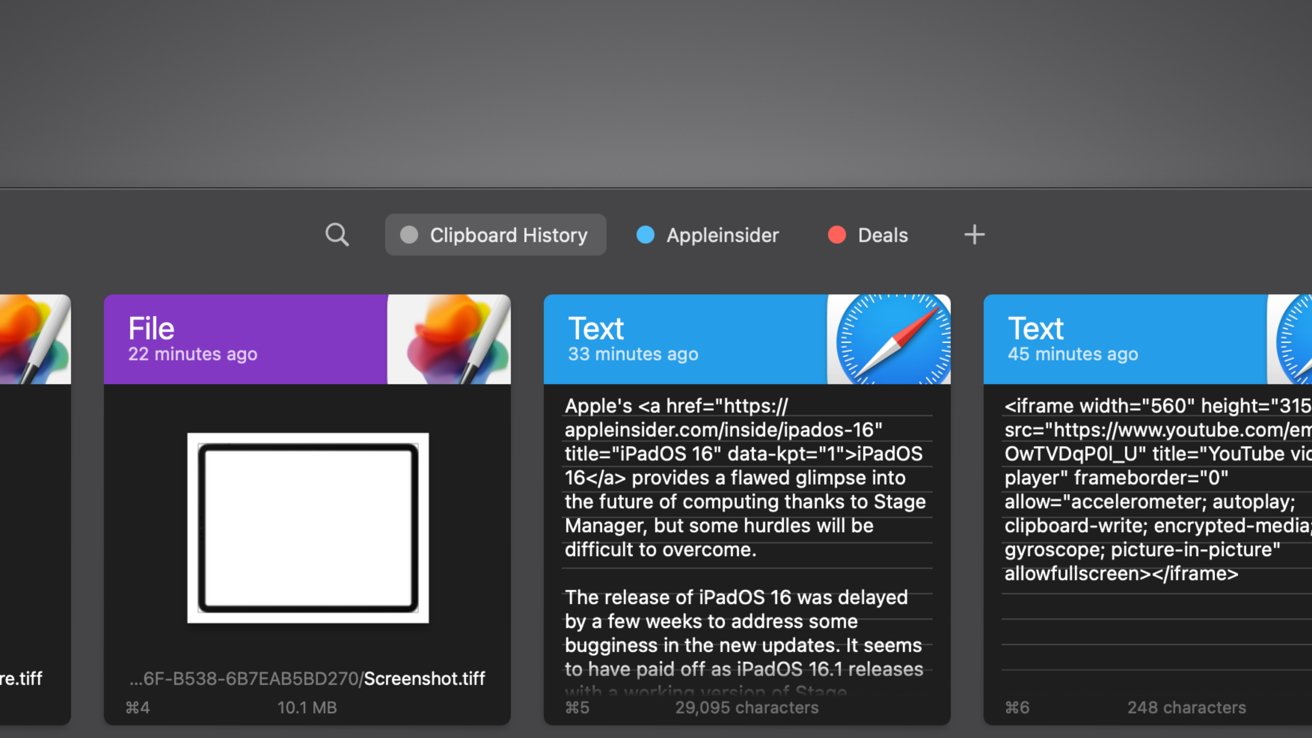The image depicts a screenshot featuring a charcoal gray background that gradually lightens toward the center. Prominently displayed in the middle is a white magnifying glass icon. Below, the text "Clipboard History" is written in white, with "C" and "H" capitalized.

Next to this text is a blue circle labeled "Apple Inc." with a capital "A," and a red circle labeled "Deals" with a capital "D." Adjacent to these circles is a plus sign. 

Further down, the display is divided into four square sections, though the first one is partially cut off. The first visible square has a purple banner at the top with "File" written in white text and is timestamped "22 minutes ago." In the upper right corner of this square, a graphic resembling a drawing is visible. Below this, there is a white square labeled "Screenshot.tiff."

The next square has a blue banner with "Text" in white print and is marked "23 minutes ago." This section contains the following text: "Apples provide a flawed glimpse into the future of computing thanks to Stage Manager. With some hurdles, it'll be difficult to overcome."

The final square, timestamped "45 minutes ago," also features a blue background with white text, mirroring the style of the previous text-based section.